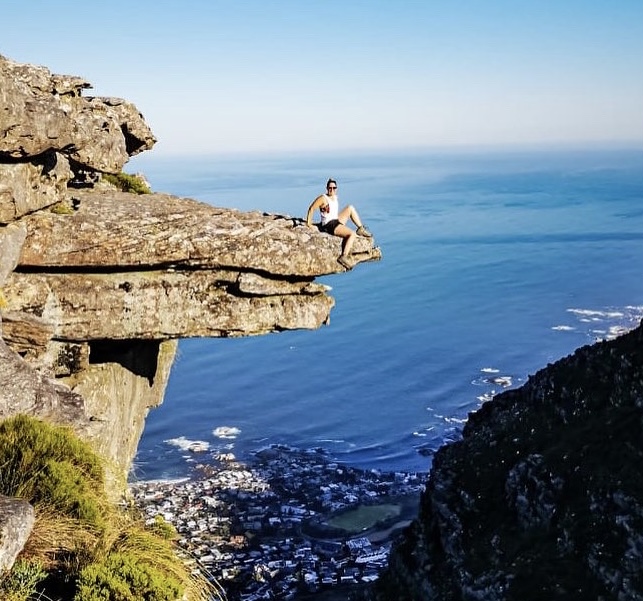This color photograph, taken outdoors during the daytime, features a stunning seaside view with a large body of water, presumably the ocean, stretching out in a beautiful shade of blue that almost blends with the sky. In the background, a small seaside village is visible along the bottom edge of the image. The photograph's focal point is a rocky outcropping on the left side, resembling a bird with its beak jutting out as a long ledge. Perched at the very tip of this high, craggy ledge is a woman sitting on the edge of the cliff. She is wearing what appears to be black shorts and a white shirt, though the distance makes specific details fuzzy. With her right leg dangling over the edge and her left leg bent upwards in a V shape, she steadies herself with her hands resting behind her on the rocky ledge. She gazes directly at the camera, smiling, capturing a moment of serene thrill high above the ocean with a vast, uninterrupted view.